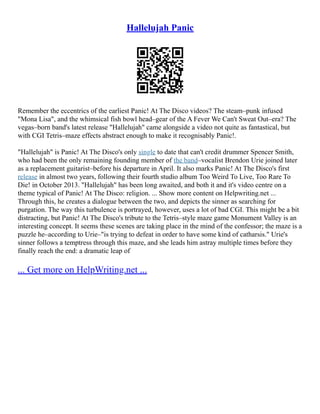The image displays a textual layout prominently featuring a QR code positioned centrally. At the very top, in blue, underlined letters suggesting a hyperlink, it says "Hallelujah Panic." Below the QR code, a detailed paragraph begins with black text, reading, "Remember the eccentrics of the earliest Panic! at the Disco videos, the steampunk-infused Mona Lisa, and the whimsical fishbowl headgear of the 'A Fever You Can't Sweat Out' era?" Continuing, it describes the Vegas-born band's latest release, "Hallelujah," which includes a video featuring CGI Tetris-mayor effects, maintaining the band's distinct abstract style. Following this paragraph, the text extends into an extensive description. At the bottom left, another blue, hyperlinked text reads, "Get more on HelpWriting.net..." The color scheme of the image includes white, black, and blue.